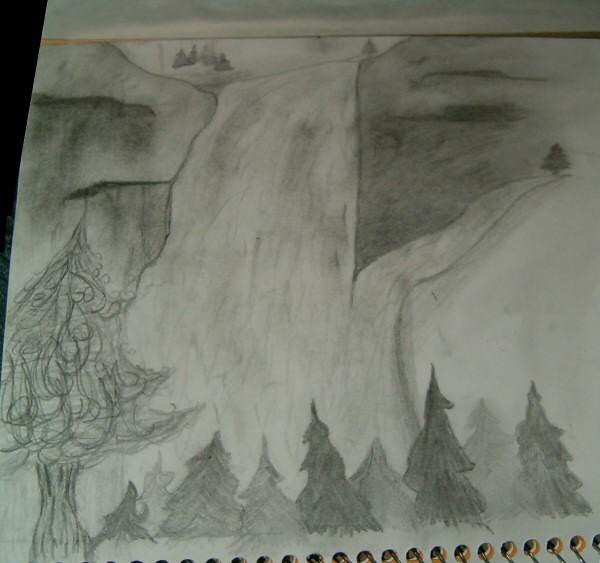This photograph captures a detailed, hand-drawn pencil and charcoal scene sketched on a piece of notebook paper. The drawing itself is held at an angle, with the top left corner of the page curving slightly away from the viewer, creating a visible black space on the left. The bottom edge of the paper reveals the presence of holes and metal rings, indicating it was created in a ring-bound notebook.

The artistic scene depicts a tranquil woodland setting with a variety of pine and evergreen trees shaded intricately at the bottom. Dominating the left side of the foreground is a large, prominent tree, providing a sense of depth. The upper section of the drawing appears to illustrate rugged cliffs or a cascading waterfall, with what seems to be ships navigating toward the waterfall, adding an element of dynamic movement. In the distance, another smaller tree is visible, further enhancing the sense of perspective. The entire scene exudes a serene yet dramatic atmosphere, skillfully rendered in rich pencil and charcoal textures.